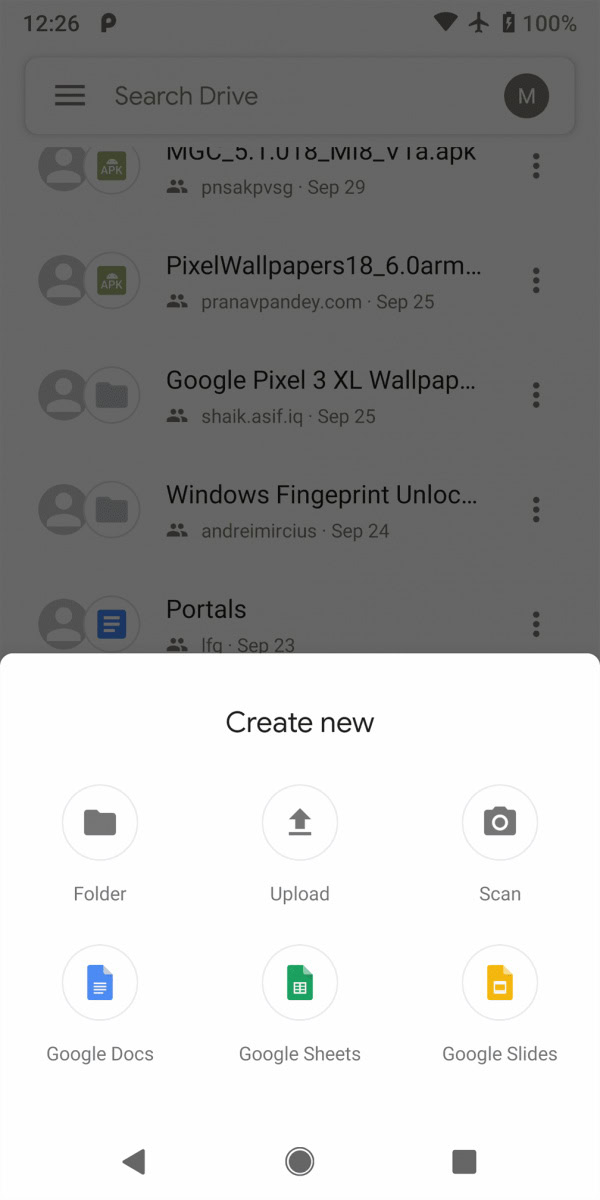The image is a screenshot from a mobile phone, showcasing a combination of a dimmed interface with a prominent pop-up towards the bottom. The top half of the screen is greyed out, indicating an overlay or a background blur effect. In this area, the status bar displays the current time, 12:26, on the upper left, alongside icons for Wi-Fi, airplane mode, and a fully charged battery on the upper right.

Beneath the status bar is a "search drive" function, followed by a list of search results featuring small round user icons to the left of each item. The displayed search results include partial text and file names such as "pixel wallpapers," "18_6," "DARM," "Google Pixel 3XL wallpaper," "Windows fingerprint unlock," and "portals," which is associated with a small blue icon, likely representing Google Docs. The first item in the list is partially cut off and unreadable.

At the bottom portion of the screen is a prominent white pop-up box with a slightly curved edge. This box appears to offer options to create new items. At the top of the pop-up box, there's text that reads "Create new." Below this header are a series of icons encircled and labeled, including a grey folder icon, an upload icon, a scan icon, a camera icon, a blue Google Docs icon, a green Google Sheets icon, and a yellow Google Slides icon.

Finally, at the very bottom of the screen, the phone's navigation bar is visible, featuring a black back button, a home button in the center, and a square recent apps button on the far right.

This detailed screenshot captures the user's interface when interacting with Google Drive on a mobile device, highlighting both file management options and the creation of new documents.